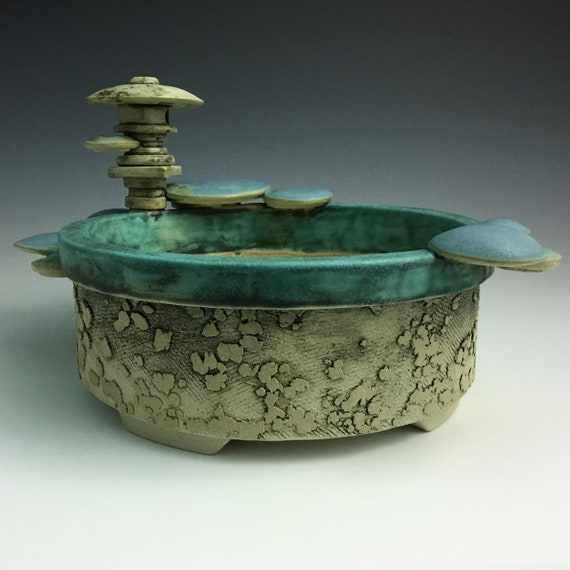This full-color, vertically rectangular, staged photograph, set indoors with artificial lighting, features a unique and intriguing arrangement. Dominating the scene is a possibly metal or ceramic bowl with a turquoise-green hue and a brown bottom, adorned with intricate relief-like markings resembling clout elements on its side. Inside this bowl sits a smaller, dark green bowl positioned toward the right. Strikingly, at the top left-hand corner of the composition, there's an enigmatic metallic object resembling a small tower with a mushroom-shaped top, a neck, and a base, all placed on the lip of the larger bowl. Additionally, two circular green dishes rest on the edge of the main bowl. The background gradient transitions from a very white bottom to a dark gray top, offering a stark contrast that highlights the unique color palette and odd shapes within the scene.